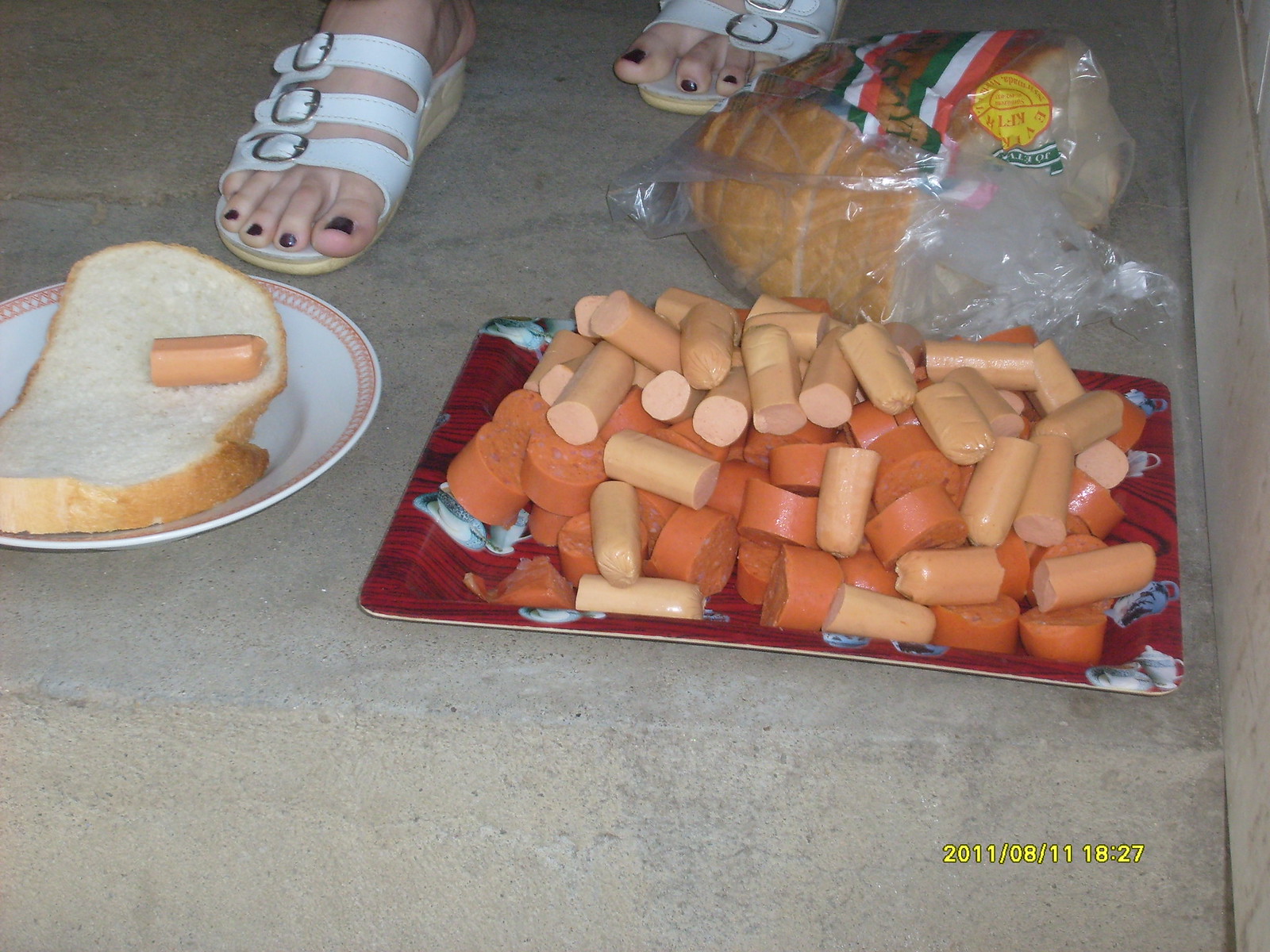This color photograph, dated 2011-08-11 at 18:27, depicts a food scene on a cement floor. A woman's feet, adorned with white sandals featuring three straps and silver buckles, with toenails painted a dark maroonish color, are visible near the food. On the ground in front of her feet, there is a rectangular red tray with a printed design, holding an array of cut-up hot dogs and sausage pieces, varying in pale yellow and reddish hues. To the left of this tray, a white plate with a pink rim holds a long slice of bread topped with half of a light-colored hot dog. Positioned behind the food items is a partially opened plastic bag containing a loaf of sliced bread decorated with an Italian flag design. The setting appears to be an outdoor or possibly industrial area characterized by a concrete floor and wall.